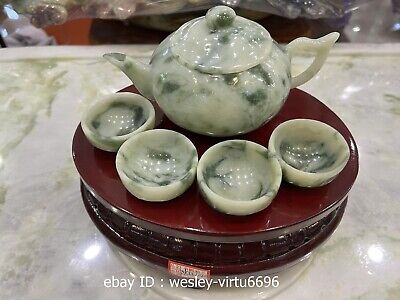The image depicts an elegant tea set arranged meticulously indoors on a highly reflective white marble surface with subtle green patterns, enhanced by overhead lighting. At the center is a cream-colored teapot adorned with olive green flecks, accompanied by its four matching teacups. These vessels are placed on a small, dark, reddish-brown mahogany turntable, contrasting the marble tabletop. The background includes various blurred objects, emphasizing the focus on the sophisticated tea set, designed perhaps for savoring green tea, given its traditional aesthetic.